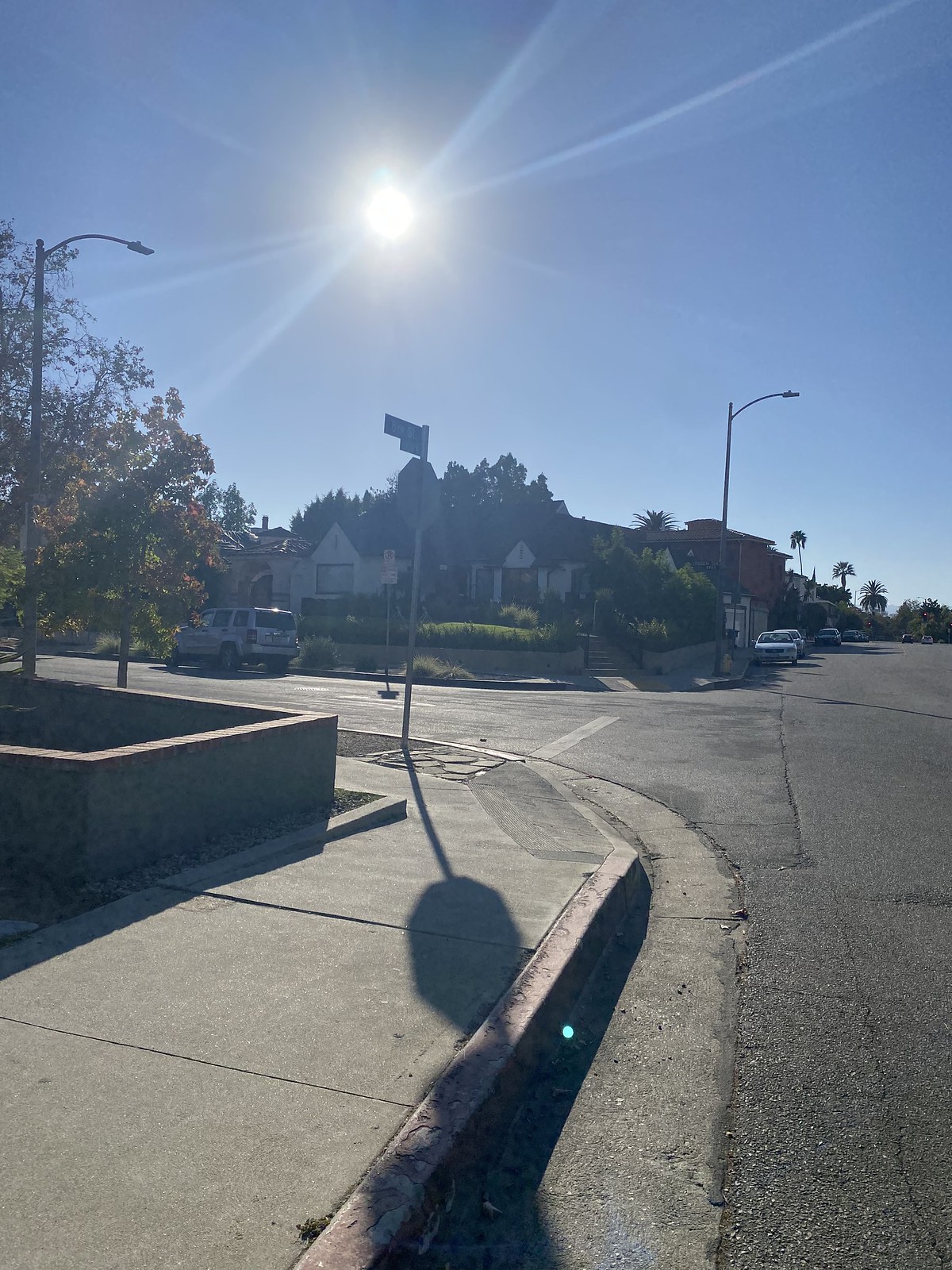In this realistic photograph, a radiant blue sky forms the background, dominated by a brilliant white sun whose distinct rays fan out from the center, illuminating the scene. Below this celestial display, a gray paved road starts in the lower right corner of the image and extends into the distance, curving to the left. Tall palm trees line the sidewalk on the left side of the road, with a few cars, including a noticeable silver one, parked along the curb. Adjacent to the intersection stands a charming house with a triangular-shaped, black roof. At the corner of the intersection, the back of a tall stop sign and two shadow-covered green street signs are visible. The lower left corner of the photograph captures part of the sidewalk bordered by verdant bushes, a lamppost, and several trees, adding to the serene and sunny suburban vista.